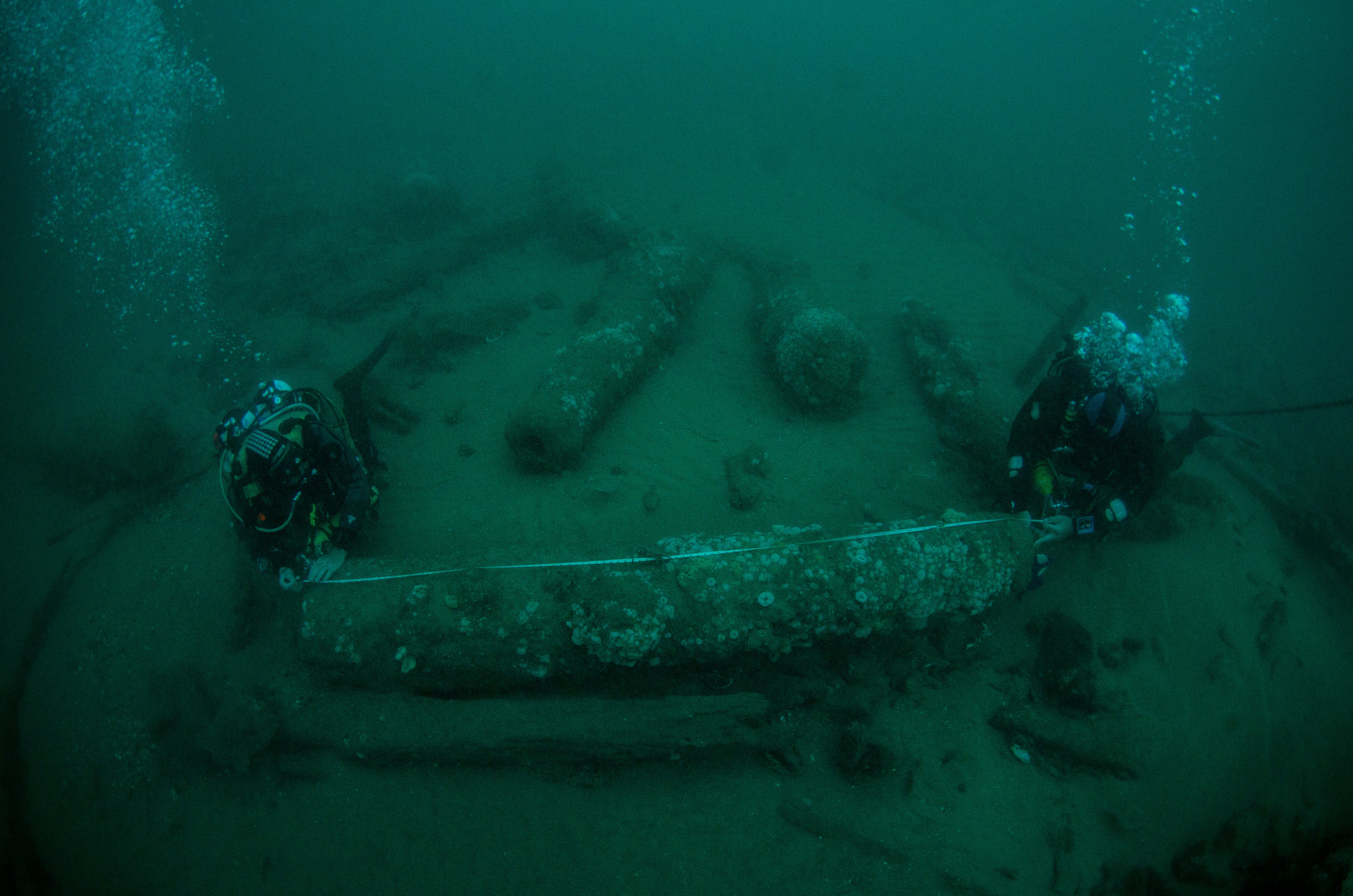In this underwater photograph taken at the bottom of the ocean, two scuba divers are positioned on the left and right sides of the image, facing the camera head-on. Both divers are fully equipped in scuba suits, and air bubbles can be seen rising from their heads. They are each holding opposite ends of a measuring tape and are focused on measuring a long, rectangular object that lies between them on the beige sandy ocean floor. This central object appears to be a column or a pipe, heavily encrusted with moss and white barnacle growths. The water is a murky green-blue, giving the scene a deep underwater appearance. Surrounding the divers are multiple oblong-shaped objects scattered across the seafloor, resembling logs or additional columns, also covered in moss and barnacles. Smaller stones and a piece of wood are situated in front of the main object they are measuring, contributing to the sense of debris and underwater ruin in this dark, murky environment.